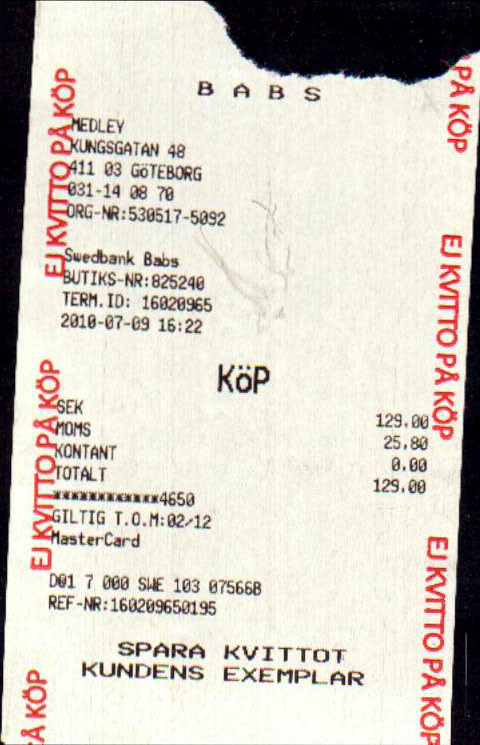This vertical rectangular image displays a slightly torn, grayish-white sales receipt against a black background. At the top center, in black all-caps text, it reads "B.A.B.S." The sides of the receipt feature vertically printed red text repeating, “E.J. Cavito Pay Cop,” on both edges. The main section of the receipt includes left-aligned black text listing transaction details: it mentions the location "Medley, Kungsgarten 48, 4-11-03, Göteborg," along with a series of numbers "0-3-1-1-4-0-8-7-0." More details follow under "Swedbank BABS" with additional numerics, indicative of a financial transaction. The receipt also specifies the total amount spent was $129 on two items, confirmed to be paid with a MasterCard. The bottom of the receipt contains centered text: "Spara Kvitot," and below that, "Kundens Exemplar." Towards the bottom are also typical credit card receipt details such as a bank name, an account number, term ID, date, time, subtotal, and a reference number.